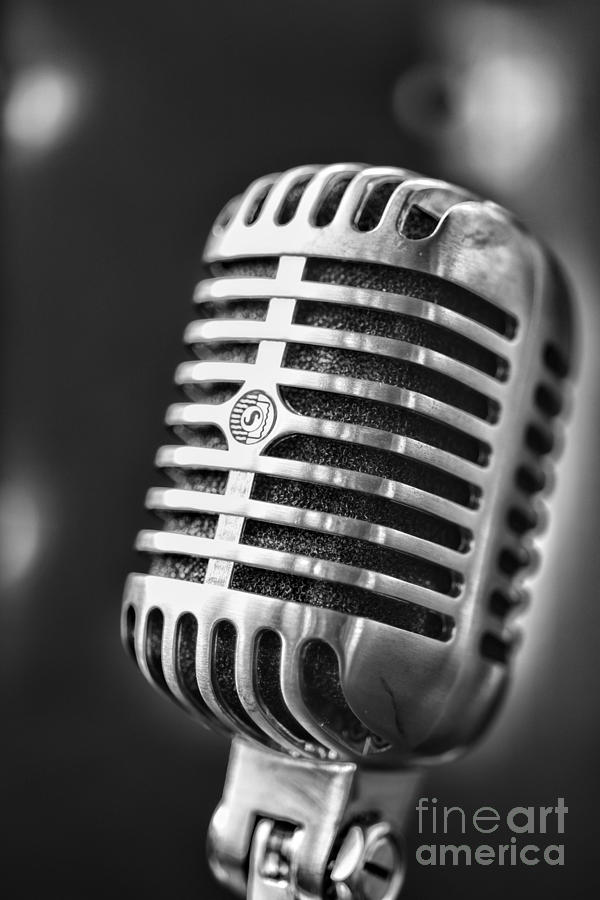This is a close-up photograph of a vintage-style, silver microphone, prominently featuring an "S" emblem. The microphone, characterized by its seven horizontal metal strips and vertical graded design across its face, is the central focal point, clear and brightly detailed. A black foamy mesh is visible behind the metal strips, enhancing its classic look. The microphone is angled slightly towards the right, giving it a dynamic presence in the foreground. The background is a soft, out-of-focus gray with subtle hints of lighter spots, almost like distant, faded lights. The image bears a watermark in the bottom right-hand corner that reads "Fine Art America," indicating the likely source. The entire photograph has a monochromatic palette, emphasizing blacks, grays, and silvers, creating a timeless and realistic aesthetic, reminiscent of old radio broadcasting equipment.